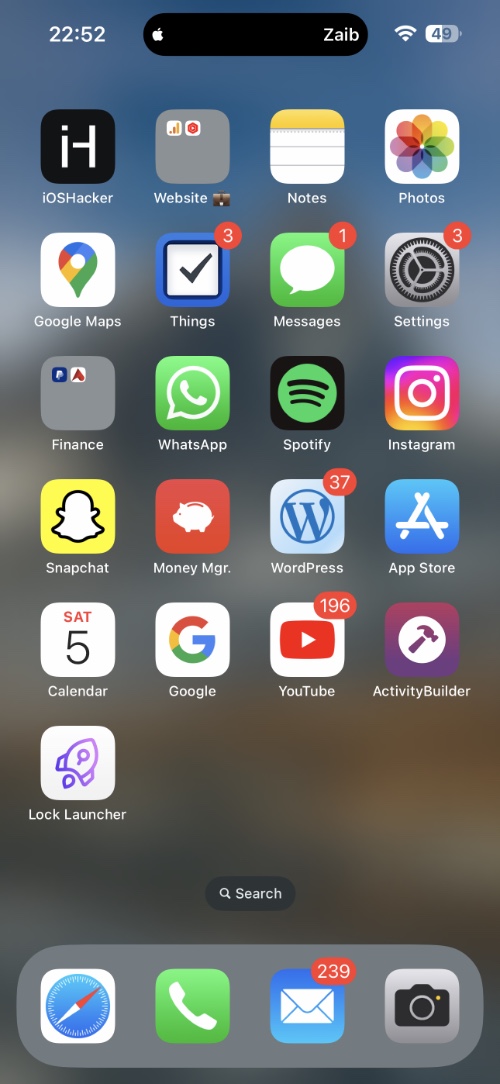The image depicts the main home screen of an iPhone, identifiable by the presence of the Safari app at the bottom. There are four primary icons stationed at the bottom dock. The first icon is Safari, recognizable by its distinctive compass logo with a blue background and a red and white needle, and labeled "Safari 1." Next to Safari is the green Phone app icon, followed by the Mail app, which prominently displays a red notification badge showing 239 unread messages. The fourth icon is the Camera app.

At the very top of the screen, the status bar displays the current time in military format, 22:52. The middle of the screen features a blue, curved-edged rectangle with the label "Zob" and a small Apple icon next to it. The status bar also indicates a Wi-Fi connection and the battery level at 49%.

The home screen is organized into six rows of apps. The first five rows are completely filled with four apps each, while the last row contains only one app. The first row includes apps like iOS Hacker, Website, Notes, and Photos. The second row features Google Maps, Things, Messages, and Settings apps. The third row hosts finance-related apps such as PayPal and another with a red "A" icon, followed by WhatsApp, Spotify, and Instagram. The fourth row contains Snapchat, Money Manager, WordPress, and App Store. The fifth row, from left to right, includes the Calendar app (showing "Sat 5"), Google, YouTube, and Activity Builder. Finally, the lone app in the sixth row is Lock Launcher, depicted with a rocket icon.